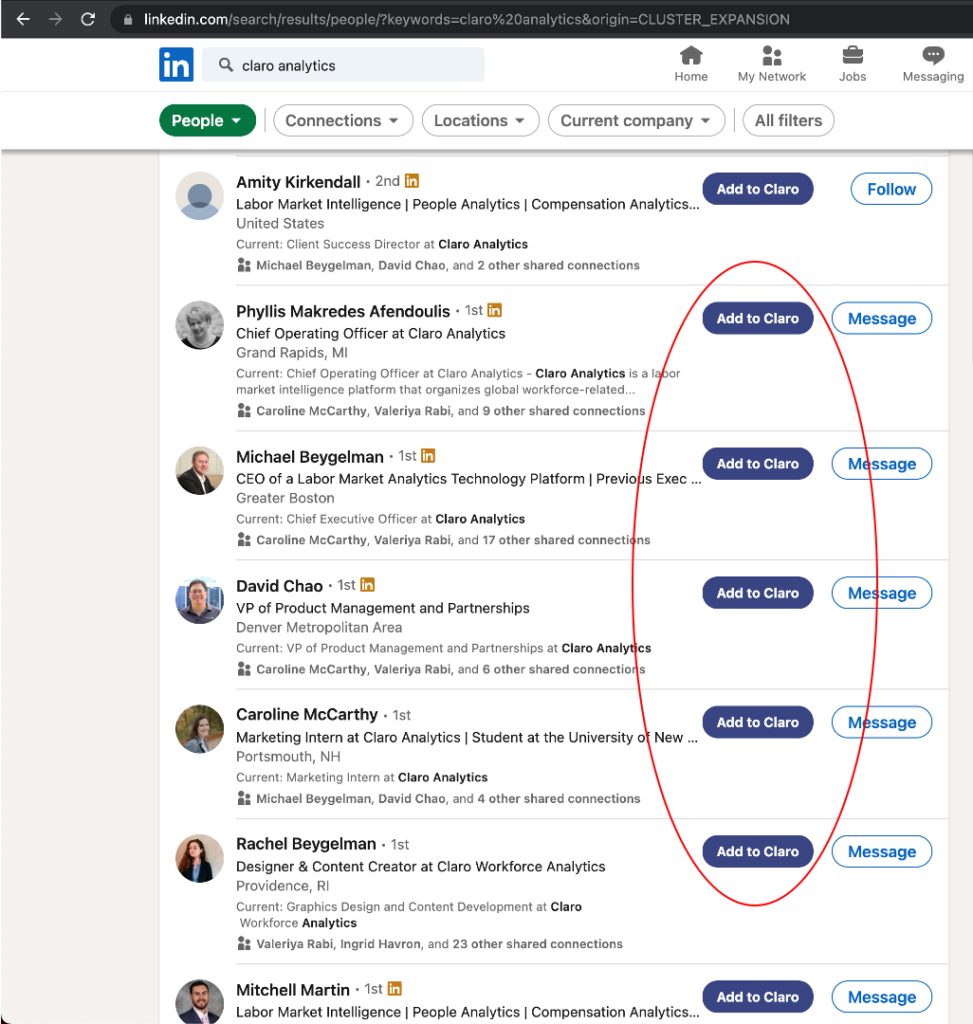A detailed descriptive caption for the image could be:

"This image depicts a screenshot from a LinkedIn.com search query for 'Claro Analytics.' At the top of the screen, a long URL is visible, indicating the specific search results page. The interface showcases the 'People' section, one of several options that also include 'Connections,' 'Locations,' 'Current Company,' and 'All Filters.' Key navigation icons are present at the top, allowing users to switch between 'Home,' 'My Network,' 'Jobs,' and 'Messaging.'

In the search results under the 'People' tab, seven individual profiles are displayed in a list. Each profile entry provides detailed information, such as the connection level (1st, 2nd, or 3rd degree), the person's location, their current job title and employer, and clickable connections. Buttons labeled 'Add to Claro' and 'Message' are available for interaction, arranged in two columns alongside each profile entry.

Notably, a red marker has been used to circle five of the central profiles, specifically the second through the sixth entries, while the first and the last entries remain unmarked."